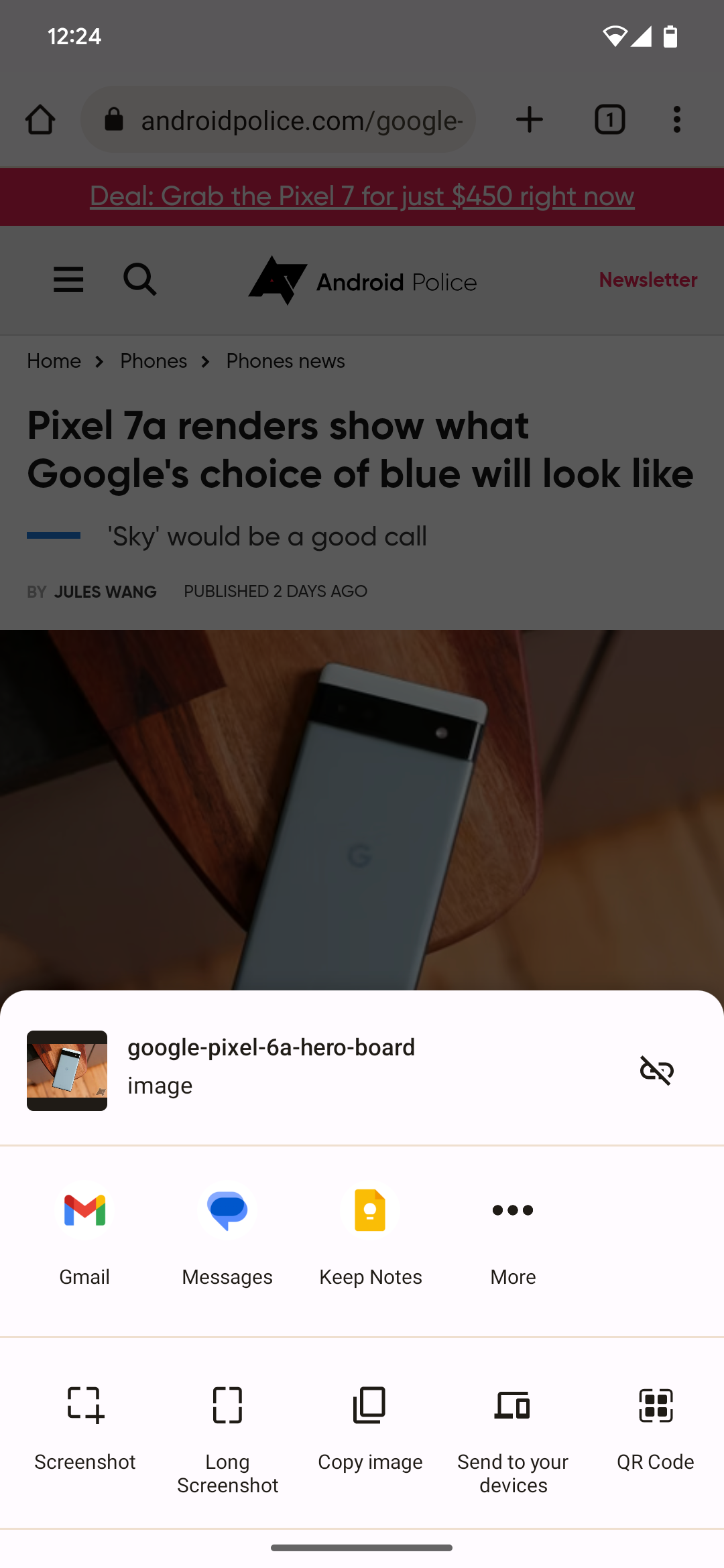This image appears to be a screenshot captured on a smartphone. The top area of the screen is notably blackened out, but faint text beneath the obscured section reads, "Pixel 7a renders show what Google's choice of blue will look like." The word "Sky" is depicted in quotes, suggesting a sky-blue color variant, and it is mentioned as "a good call." The accompanying text credits by Jules Wang and indicates the article was published two days ago on androidpolice.com. The top of the screen displays the Android Police logo, alongside typical smartphone indicators such as battery life, a triangular warning icon, and Wi-Fi connectivity status. 

As the image continues downward, it references "Google pixel/Google-pixel-6a-hero-board-image," likely pointing to a related image or section within the content. Various application icons are visible, including an 'M' for Google Mail, a speech bubble for messages, an orange box for Google Keep Notes, among others. The user interface options shown include features like 'Screenshot,' 'Long Screenshot,' 'Copy Image,' 'Send to Your Devices,' and a QR code.